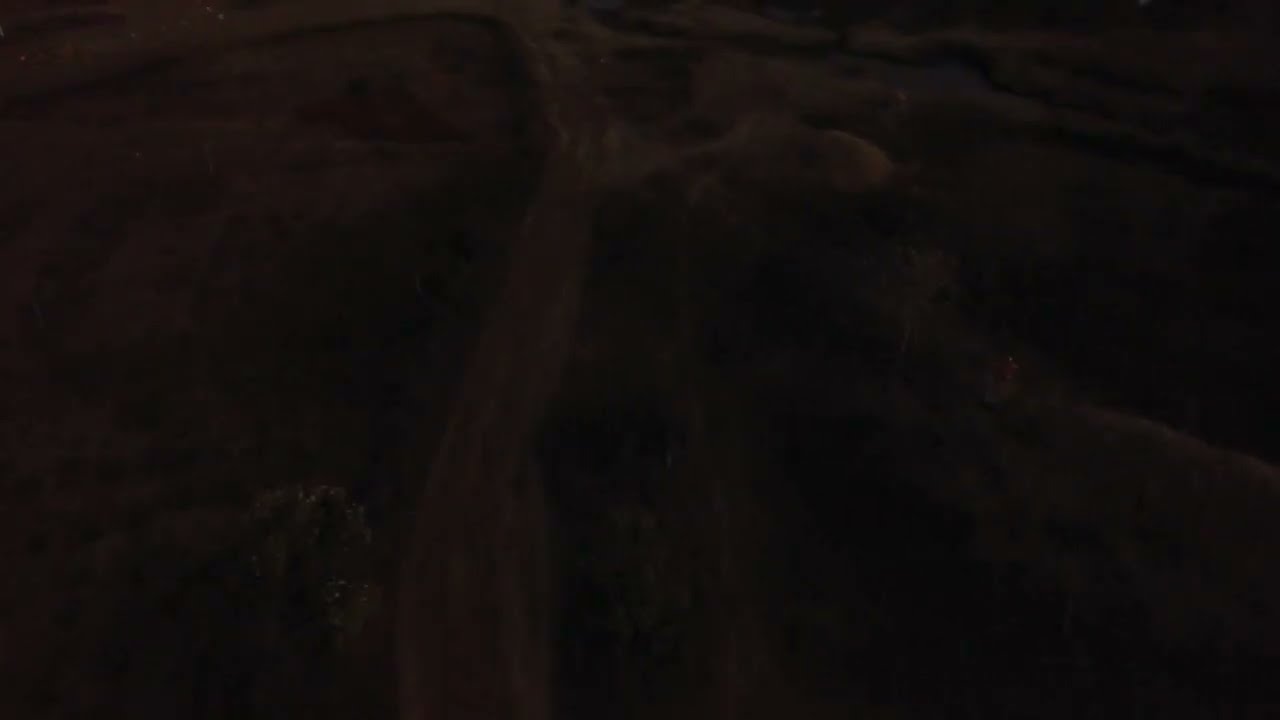The image is an extremely dark photograph, predominantly solid black, making objects difficult to discern. Upon closer inspection, just to the left of center, a tree formation emerges. This tree, dark brown in color, originates from the bottom of the image and ascends towards the top. Near its upper sections, the tree splits into branches extending left and right. Sparse green vegetation adorns the tree, but the darkness makes it hard to notice. To the right of center, near the top, another lighter brown section of the tree becomes visible, surrounded by hard-to-see green vegetation.

The rest of the image is overwhelmingly black, particularly in the upper right, bottom right, and bottom left corners, as well as the left upper corner, where no discernible details can be made out. The landscape appears to be viewed from an elevation, possibly showcasing a flat field common to farm areas. Extending from the bottom edge of the image is a dirt road stretching forward to the top edge. Near the top, this pathway forks to the right, continues straight, and curves slightly to the left. A small dust cloud can be seen billowing up from the area just to the right of the fork.